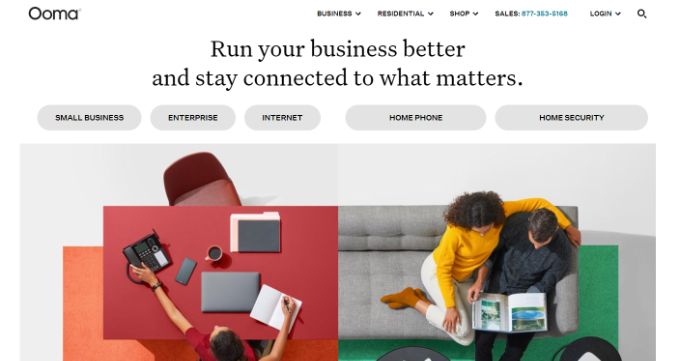**Detailed Caption for the Image:**

This image is a screenshot of a website with a clean, white background and no visible border. At the top left corner, the text "OMA" is displayed, while the top right corner features navigation options: "Business," "Residential," "Shop," "Sales," "Login," and a search icon resembling a magnifying glass. Next to "Sales," a blue contact number, 877-353-5148, is visible. Below these navigation items, a prominent headline reads, "Run your business better and stay connected to what matters."

The webpage features five oval-shaped buttons labeled: "Small Business," "Enterprise," "Internet," "Home Phone," and "Home Security." Below these buttons, there are two interconnected images. 

The first image on the left shows a bird’s-eye view of a person seated at a red desk. On the desk, there is a landline phone, a cup of coffee, several folders, a closed laptop, and the person appears to be writing in a book or notebook. The second image to the right shows a top-down view of two individuals sitting on a couch. They are engaged in reading or looking through a book or magazine together. The couch is positioned adjacent to the desk from the first image, creating a cohesive visual blend between business and personal environments.